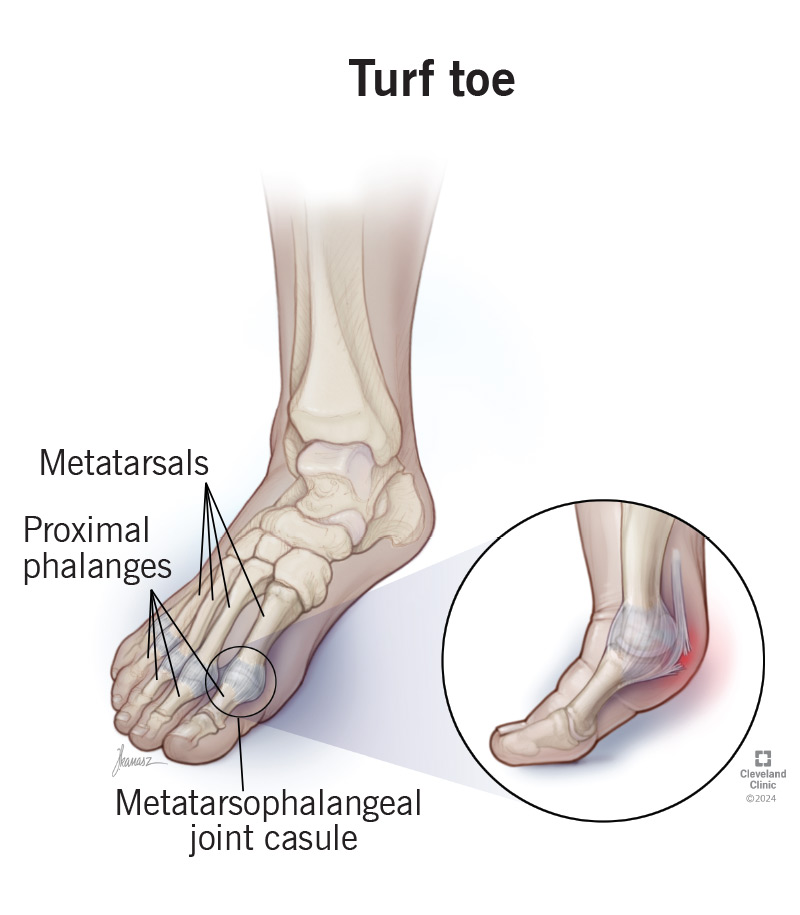The illustration, resembling a high-quality, computer-generated image typical of a college textbook or Google resource, explicates the condition known as "turf toe." Set against a white background with bold black lettering at the top spelling "turf toe," the left side of the image prominently features a detailed depiction of a foot and lower shin. The bones within the foot, illustrated in shades of brown, are meticulously labeled. Four lines extend from the term "metatarsals," indicating these long bones. Beneath this, another set of arrows points to the "proximal phalanges," highlighting the toe sections. Further below, the "metatarsophalangeal joint capsule" is specified with illustrative lines converging on the major joint of the big toe where bending occurs.

Adjacent to this primary depiction, a circular inset on the lower right provides a close-up side view of the big toe. This zoom-in vividly portrays the metatarsophalangeal joint capsule appearing torn, red, and inflamed, indicative of injury. The entire image is accompanied by a small trademark in the lower right corner, stating "Cleveland Clinic, 2004," ensuring its authoritative source.